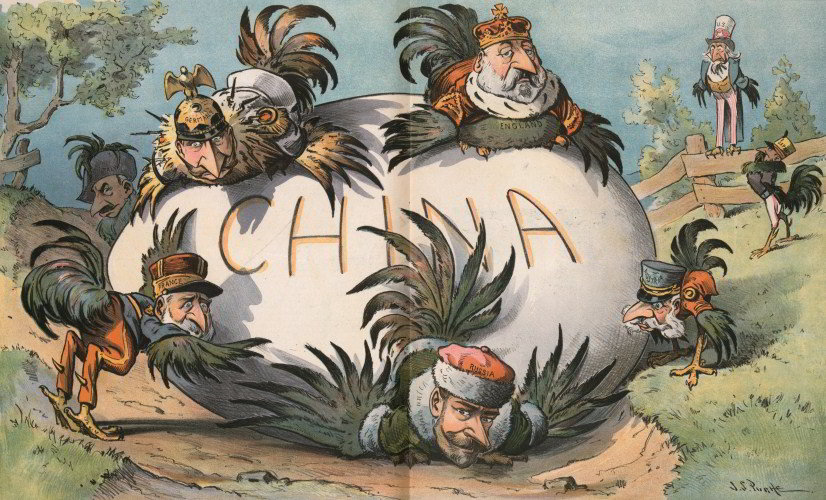The image, resembling an illustration from a book or magazine with a visible fold down the middle, depicts a large white egg with "China" written on it in black letters outlined in yellow. The egg is central to the scene, crushing a man wearing an orange hat with white fur trim, labeled "Russia." Atop the egg sits a figure with a bird-like body, crowned and adorned with a fur collar, labeled "England," with feathers featuring human faces. To the left is another bird-like figure with a helmet that has an eagle insignia, labeled "Germany." On the left side of the egg is a figure with "France" on his hat, pushing the egg, and to the right, although less clear, possibly a figure representing Japan. In the background, a character in an Uncle Sam hat, representing the USA, stands on a wooden fence, observing the scene. The landscape includes trees, dirt, and grass under a blue daytime sky, completing the detailed satirical portrayal of international relations.